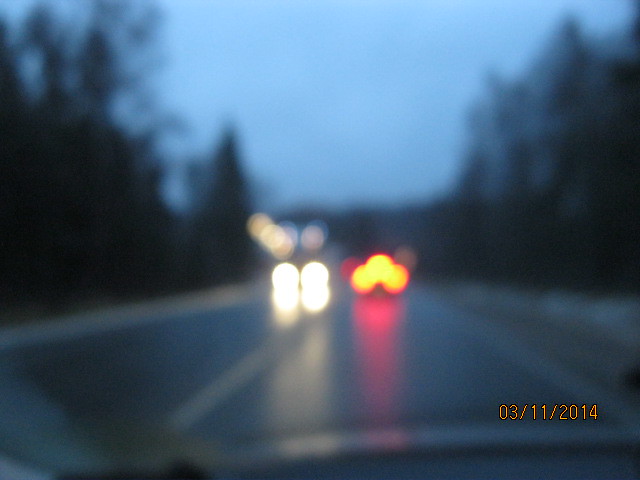A photograph captured from inside a vehicle reveals a scene unfolding during either dawn or dusk, possibly on a stormy day, given the subdued lighting. In the bottom right-hand corner, a timestamp reads "3-11-2014," indicative of a camera or phone's photograph. The image is taken from the dashboard perspective, portraying the road ahead. White headlights from an oncoming vehicle pierce the semi-darkness, while the taillights of the car directly in front cast a warm glow. The sky overhead is a moody, dark grayish-blue, suggesting an overcast or rainy atmosphere. The wet street below reflects the glistening headlights and taillights, enhancing the scene's dramatic effect. Flanking the road on both sides are tall, shadowy trees, adding depth and a sense of seclusion to the image.